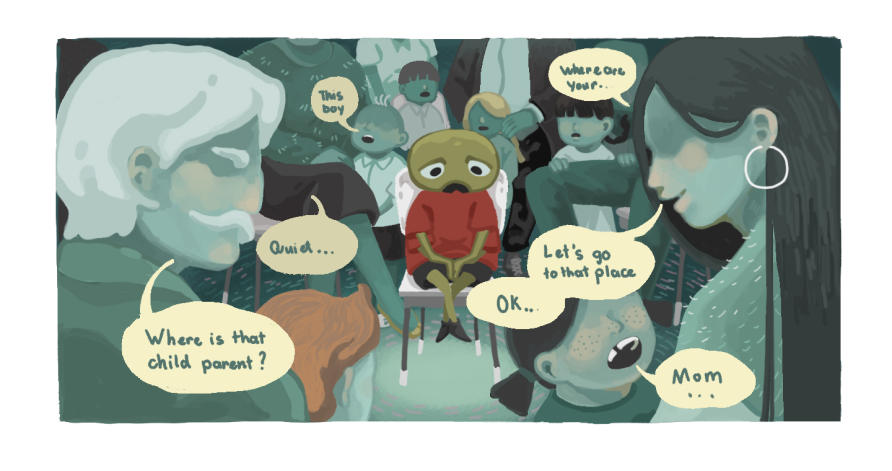In this detailed artistic sketch reminiscent of a graphic novel or comic strip, children are seated in chairs at the center of the scene, their figures rendered in fine detail. Dominating the middle is a peculiar child with bald, olive-toned skin, striking dark eyes, and a downturned black mouth, dressed in a red shirt and black shorts with bare legs and black shoes. 

To the left stands a man with long, white hair, a matching mustache, and eyebrows, captured with a light beige facial tone. A speech bubble emanates from his mouth, asking, "Where is that child's parent?" Below his mustache, another's voice demands, "Quiet." 

On the right, a woman with long hair adorned by a prominent hoop earring is depicted in profile. Her speech bubble suggests, "Let's go to that place," while a nearby child, mouth agape, cries out, "Mom." In the background, another child points out the central figure, exclaiming, "This boy."

The entire illustration conveys an eerie, possibly disquieting, atmosphere enhanced by the enigmatic expressions and the surreal conversations that frame the unusual, olive-skinned child at the heart of the image.